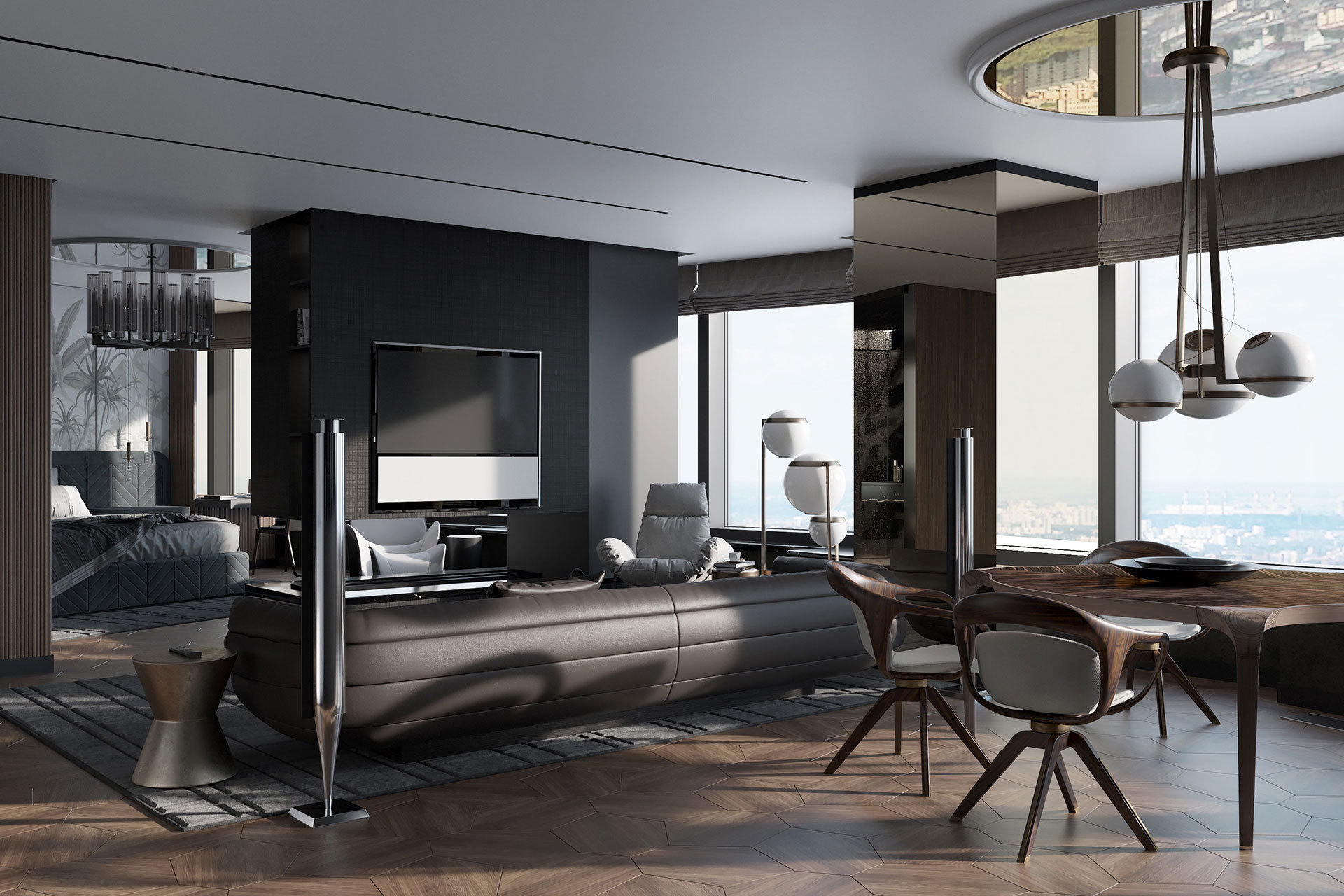This image captures the interior of a modern living room and dining area bathed in daylight, showcasing a chic, contemporary design. The space features expansive glass windows on the right side, providing a panoramic view of a blue sky, possibly overlooking an ocean. The room is dominantly decorated in dark neutral tones with a mix of browns, off-whites, and blacks.

Centering the aesthetic, the main living area includes a low-backed brown couch facing a black-painted wall, which is adorned with what seems to be either a large TV or a painting framed in gray and white. Adjacent to this setting, an adjoining room with a strikingly large chandelier and reflective glass elements hosts a circular brown dining table surrounded by dark wooden chairs with white cushioning. Below, the geometric patterns of the brown wood flooring add warmth to the monochromatic palette.

Hanging from the white ceiling, various off-white lamps and an ornate chandelier illuminate the room. The design seamlessly merges the living space with the dining area, emphasizing the modern, yet cozy ambiance through its strategic use of colors and sophisticated furnishings.